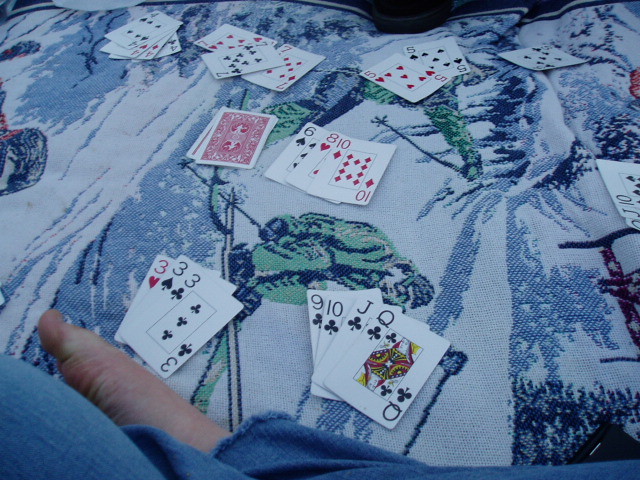In this image, a collection of playing cards is spread out on a blue and light blue bedspread with green accents. At the center of the arrangement, there are prominently displayed cards with values of 6, 8, and 10. Notably, all cards are Bicycle brand with distinctive red backs. In the foreground, we see a variety of cards including the 9, 10, and Queen of Clubs, as well as a Jack. To the left of this group are three 3's. Scattered across the bedspread in the background, there is an assortment of cards, with a cluster of 4's, three 7's, a 5, and an 8. There are also people visible in the image, seemingly playing a card game. One person, partially visible, appears to be running, and another is seated towards the far right. The bedspread's pattern underneath them appears to depict a skiing scene. The people in the image are focused on the game, having successfully matched up their cards. The cards are rendered in bold letters, making the numbers and suits easily readable.